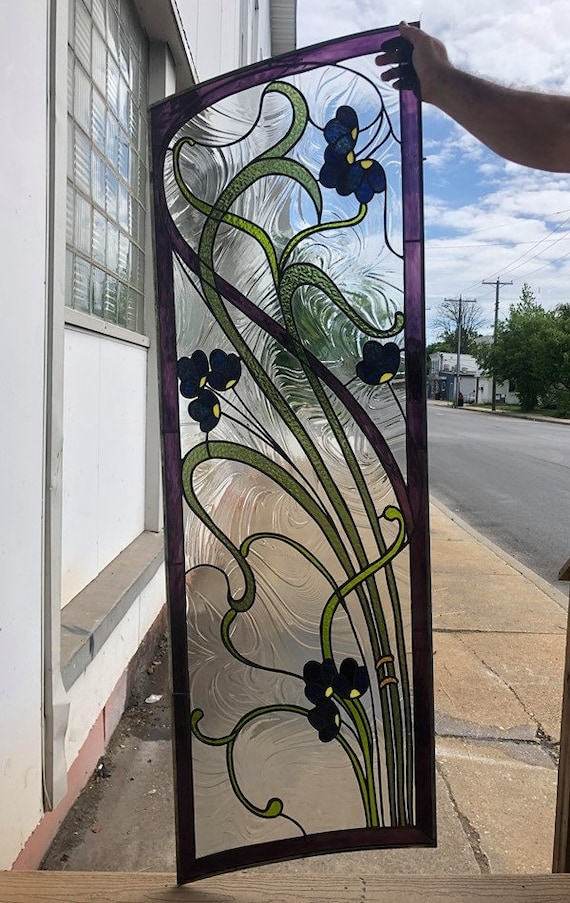This photograph captures an art piece, potentially a window or decorative glass door, held by a male hand visible at the top right of the image. The rectangular frame of the piece is metallic, colored in greyish-black. It features a central glass panel adorned with an artistic floral design. This design is detailed with green vines, purplish and black petals, and a combination of yellow and black centers for the flowers, complemented by a purple border. The artwork is positioned outdoors on a rough, tiled pavement next to a street, which runs along the right side of the frame, while to the left stands a white building with upper glass windows. The cloudy sky in the background hints at an overcast day, contributing to the urban, artistic setting of the photograph.